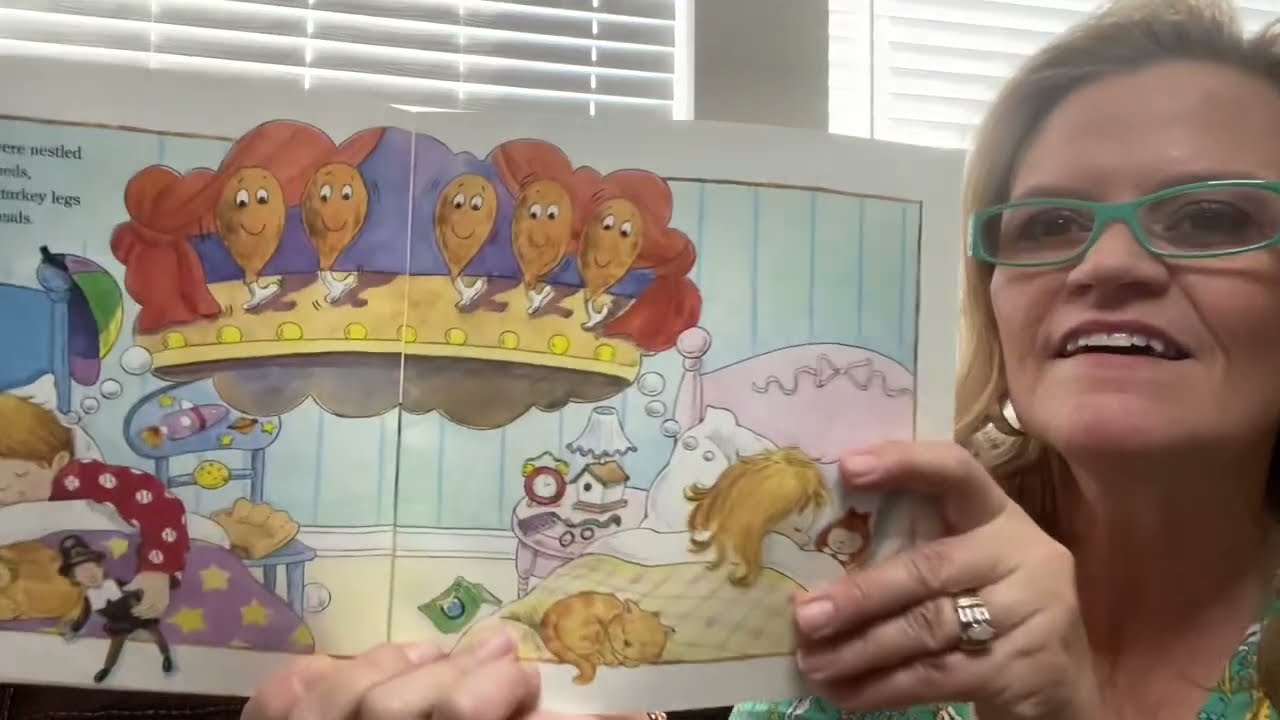In this image, a middle-aged woman with green-rimmed glasses and blondish hair, wearing a green dress, is smiling warmly at the camera as she appears to read from a children's book, possibly for a YouTube video. She holds the book open with both her hands, revealing an illustration of two children sleeping in separate beds adorned with colorful bedding. On the left, a little boy with short blond hair, dressed in red pajamas, is shown holding a pilgrim doll. On the right, a little girl with long blonde hair lies in a pink bed with a cat and a doll beside her. Above the children is a shared dream bubble, depicting cartoon turkey legs with smiling faces and little feet, dancing on a stage. The text indicates that these are indeed turkey legs, reminiscent of a Thanksgiving feast. The woman's expression and the vivid illustration make the scene inviting and cheerful.